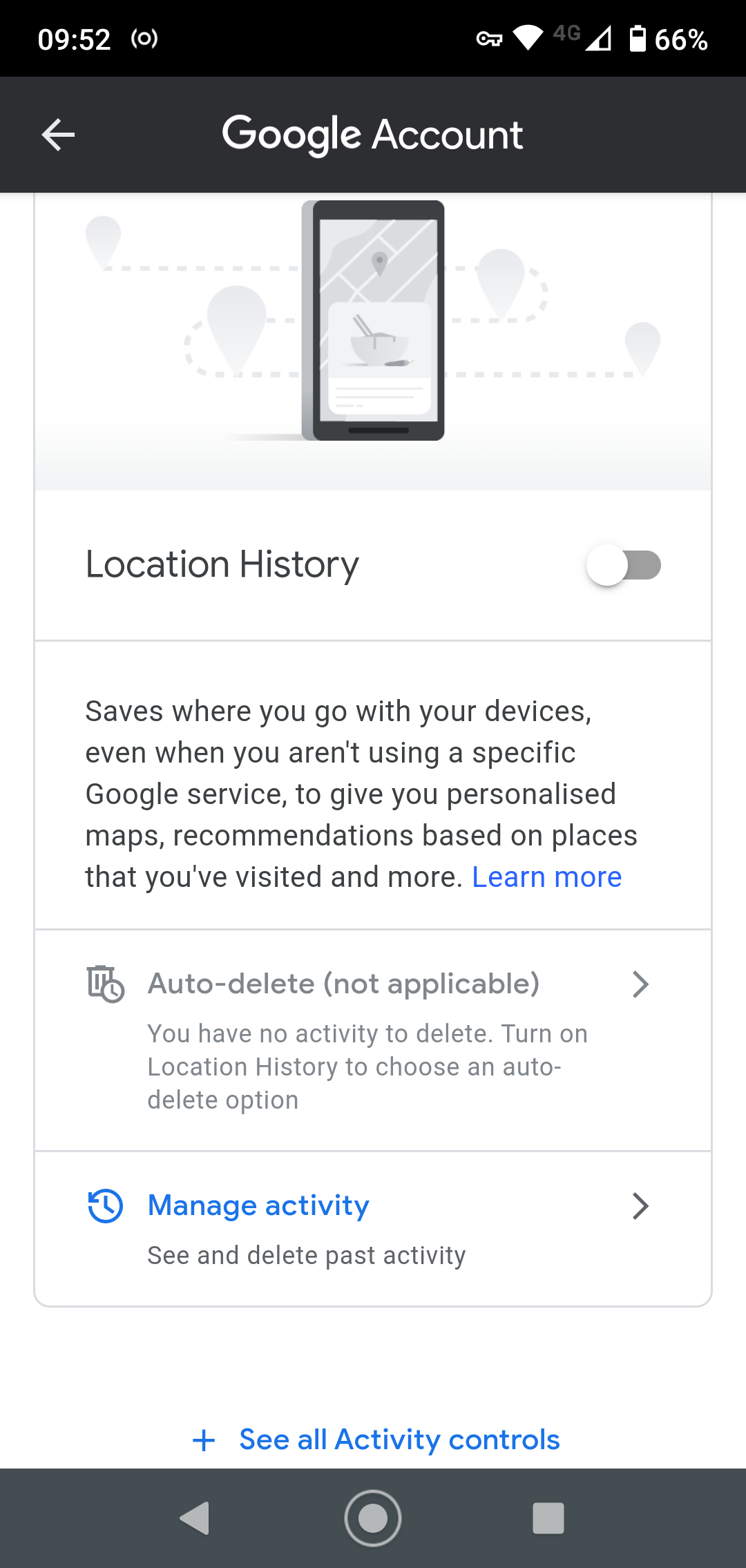This image depicts a screenshot of a section from the Google Account settings page, specifically focusing on Location History options. The screenshot is taken from a cell phone, as indicated by the status bar at the top of the screen, which displays a battery life of 66%, strong network connection bars, and the time, 9:52, positioned in the upper left corner.

The top of the image features a black header with the words "Google Account" written in white text. Below the header, there is an illustrative icon of a cell phone. Surrounding the icon are zigzag lines composed of dots, which resemble location pins in gray.

The text directly under the icon indicates that the "Location History" is currently turned off. To the right of this, a box elaborates that Location History "saves where you go with your devices, even when you aren’t using a specific Google service, to give you personalized maps, recommendations based on places you have visited, and more." There is a "Learn more" link in blue within this box.

Further down, it states "Auto-delete: Not applicable," with an arrow pointing to the right. Another message indicates that "You have no activity to delete" and suggests to "Turn on Location History to choose an auto-delete option."

At the bottom of the screen, there are two blue links: "Manage activity," which allows the user to see and delete past location data, and "See all activity controls," preceding which is a blue plus sign for emphasis.

This detailed depiction emphasizes the information and options available for managing Location History in Google Accounts, specifically highlighting how the settings can impact personalized features and data retention.